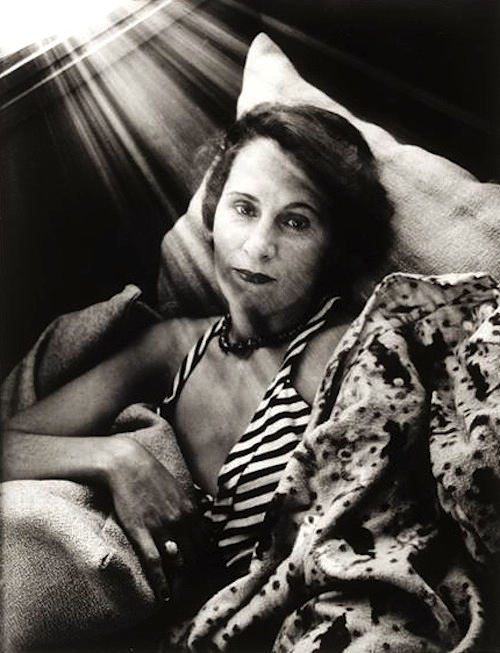The image is a sepia-toned or black-and-white photograph, possibly a very realistic painting, featuring a woman in the center. She is reclining against a pillow, with beams of light streaming in from an open window on the upper left, crossing her face. She has short, dark hair swept back and to the left side of her face, with heavy eyelids and dark eyes. She wears a dark, close-fitting necklace and a black-and-white striped halter top, emphasizing her flat chest. Her right arm is curved at the elbow, with her hand resting on a cushion in front of her. The left side of her body is partially covered by what appears to be a blanket, possibly with animal prints. The background is mostly dark, except for the radiant beams of light.